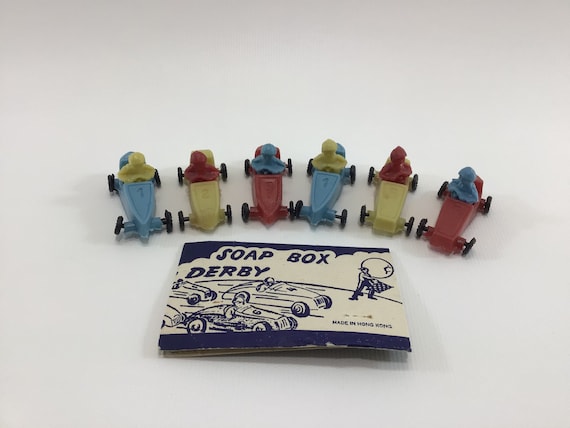The photograph features a professionally arranged collection of vintage toy soapbox derby cars. Set against a crisp, white background with deliberate lighting that casts subtle drop shadows, the image showcases six colorful miniature race cars lined up in a curved formation. Each car, made of plastic with black wheels, carries a molded plastic driver. From left to right, the sequence displays a light blue car with a green driver, a yellow car with a red driver, a red car with a blue driver, another blue car with a green driver, another yellow car with a red driver, and a second red car with a blue driver. The cars are likely numbered either one or two.

In the bottom foreground of the image sits a small white card designed like vintage packaging, marked "Soapbox Derby" in dark blue. The illustration on the card depicts stylized, old-fashioned race cars racing towards the right. The packaging adds a nostalgic touch, suggesting the cars are relics from a bygone era, possibly made in Hong Kong.